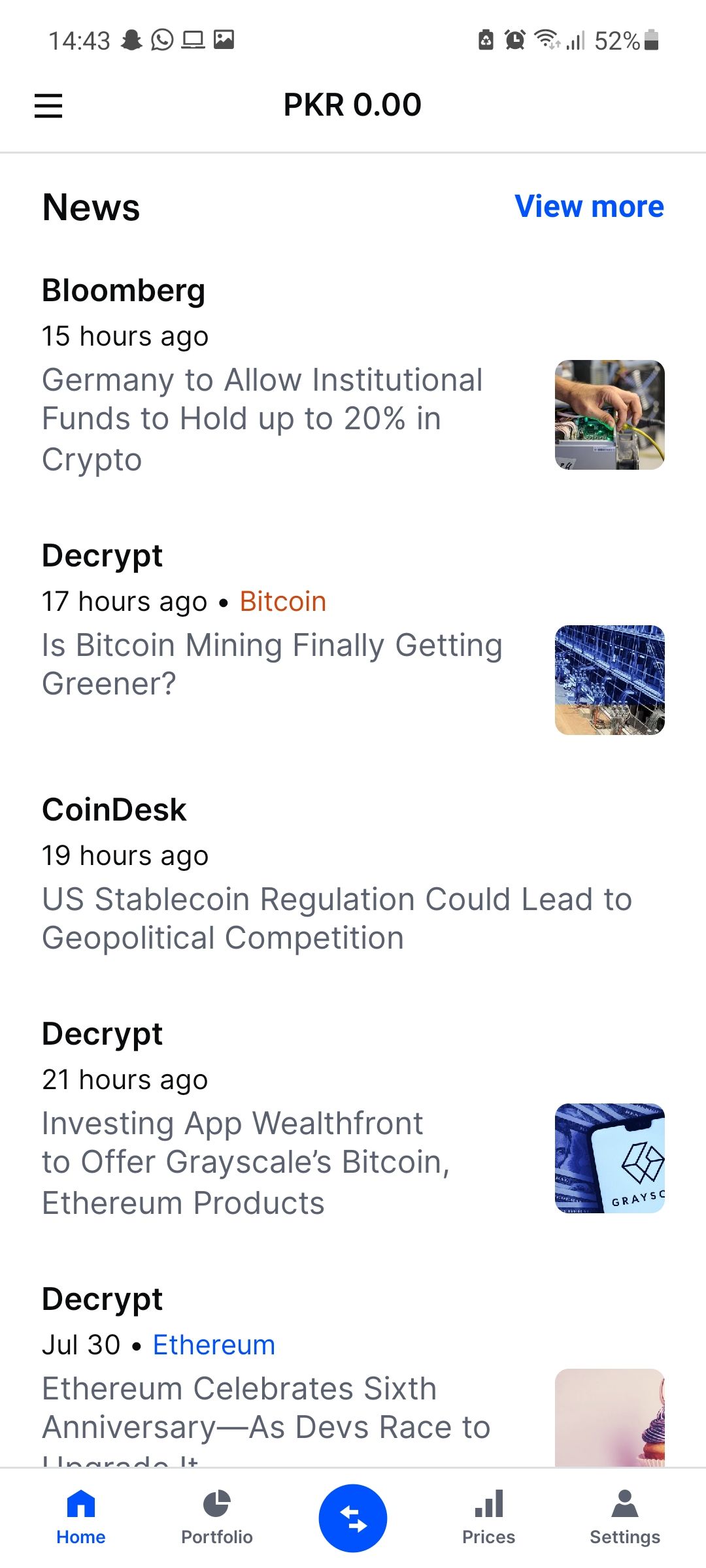**Detailed Caption for Mobile Screenshot**

The screenshot displays a mobile device screen captured at 14:43, with various app icons situated beside the time indication. On the right side of the status bar, standard status icons are visible, indicating Wi-Fi connectivity, cellular signal strength, battery life at 52%, as well as additional icons representing an SD card and an active alarm.

The image primarily shows a news application in use, featuring a clean interface with a white background and black text. At the very top of the screen, the header reads "PKR 0.0." To the left of this text, there is a menu button represented by three horizontal lines stacked in rows.

Beneath the header is a section for news, introduced by a blue link labeled "View More." The news feed is composed of various articles, each accompanied by small images on their right side. The following are the articles displayed, along with their respective details:

1. **Bloomberg (15 hours ago)**: "Germany to allow institutional funds to hold up to 20% in crypto."
2. **Decrypt (17 hours ago)**, tagged Bitcoin: "Is Bitcoin mining finally getting greener?"
3. **Coindust (19 hours ago)**: "U.S. stable coin regulation could lead to geopolitical competition."
4. **Decrypt (21 hours ago)**: "Investing app Wealthfront to offer grayscale Bitcoin Ethereum products."
5. **Decrypt (July 30th)**, labeled Ethereum: "Ethereum celebrates sixth anniversary as devs race to..." (the text is cut off).

At the bottom of the screen, navigation buttons are visible, including options for "Home," "Portfolio," "Prices," and "Settings." Centrally located is a prominent blue circle icon featuring arrows pointing in opposite directions, likely representing a refresh or sync function.

This detailed description captures the content and functionality presented in the mobile screenshot.